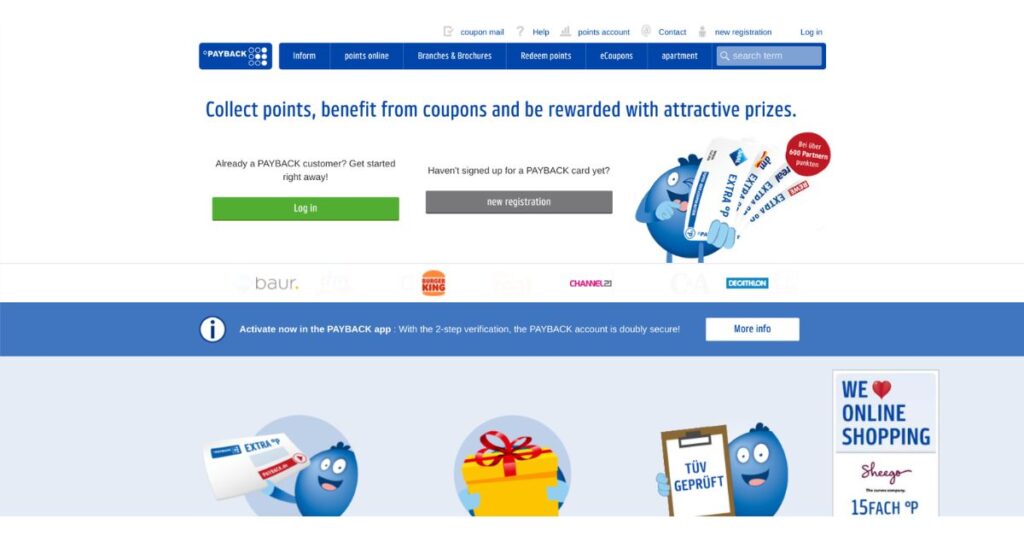The image features a website interface with a predominantly white background. At the very top right corner, there are navigation tabs which include "Coupon Mail," "Help," "Points," "Account," "Contact," "New Registration," and "Login." Beneath these, a menu on a blue background with white text offers additional navigation options such as "Payback," "Inform Points Online," "Branches and Broadcast," "Redeem Points," "E-Coupons," "Apartment," and a search bar.

The main section of the page, set against a white backdrop, contains a promotional message in blue text: "Collect points, benefit from coupons, and be rewarded with attractive prizes." Below this message, there are two call-to-action buttons with black text. On the left, a green button prompts existing Payback customers with the text "Already a Payback customer? Get started right away, login." On the right, a grey button encourages new users to register with the message "Haven't signed up for a Payback card yet? New registration." Positioned to the right of this area is a graphic of a blue emoji holding coupons labeled "Extra Op."

At the bottom of the page, there are logos for "BAUR," "Becker King," and "Channel 21." Below these logos, a blue bar with white text encourages users to enhance account security by stating, "Activate now in the Payback app with two-step verification, the Payback account is doubly secure." Accompanying this is a white button labeled "More Info."

In the lower section, another blue emoji is visible, this time holding an orange gift, a white notice board, and a newspaper or coupon. On the bottom-right corner of the image, white text reads, "We love online shopping, share, go, 15, fetch, op."